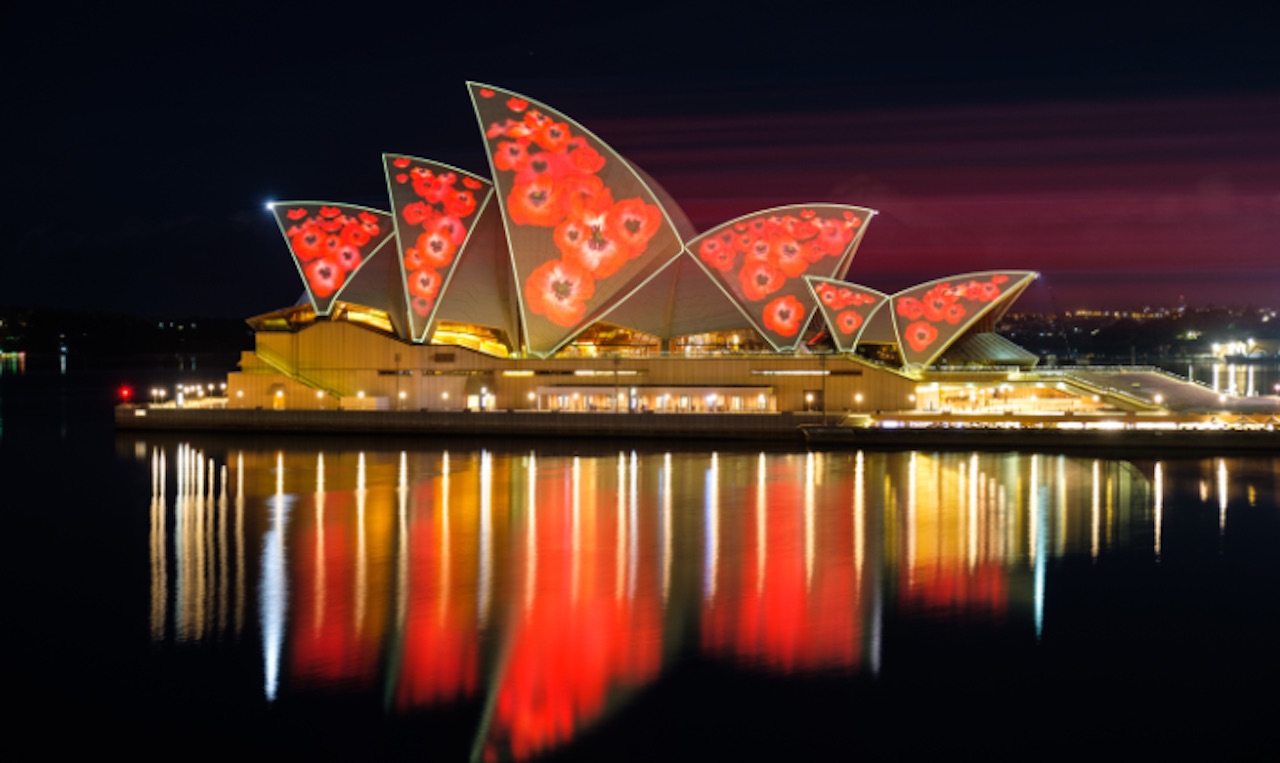This photograph captures a stunning nighttime view of the Sydney Opera House, which appears to be illuminated for a special event. The iconic sail-like panels of the Opera House are adorned with vibrant red poppy flowers featuring black centers and delicate white outlines. These floral projections transform the traditionally white structure into a shade of tan, creating a striking visual contrast against the black sky and dark waters. The Opera House is enveloped by a body of water that mirrors the vivid red, yellow, and amber lights from the building, adding to the enchanting scene. The photograph also shows tiny lit windows, contributing to the overall luminescence of the landmark. The sky above appears as a deep, blackish-purple, enhancing the dramatic effect of the illuminated Opera House against the night.